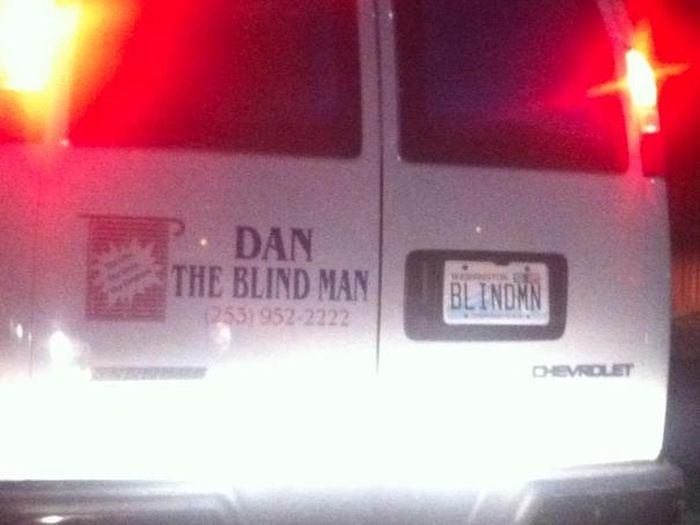This is a slightly blurry, close-up nighttime photograph of the back of a white Chevrolet business cargo van. The image shows the van from the bumper up to approximately 80% of the rear windows, which are tinted. The van's brake lights are on, and it is illuminated by headlights from another car. On the left back door of the van, there is a business logo that reads "DAN THE BLIND MAN" in large, uppercase letters, with a phone number "253-952-2222" underneath. To the left of this text, there is a visual logo featuring window blinds, and another smaller logo that is too blurry to identify. The right rear door houses a Washington State license plate, reading "BLINDMN," which aligns with the business branding theme.